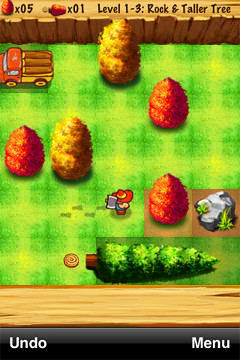The image shows a screenshot of a mobile game featuring a top-down view of a grassy field. Central to the image is a small wizard character with a red hat, white face, wearing blue pants and brown shoes. He appears to be holding an axe and is walking towards a large green pine tree, which looks like it has been cut down. Surrounding the wizard, there are three red pine cone-shaped bushes and two golden-yellow ones. There is also an orange truck with a yellowish-brown back in the upper left corner. At the bottom of the screen, a black silvery strip contains red text that reads "undo" on the left and "menu" on the right. Additionally, some game stats such as "Level 1 to 3," and indicators for "five of those and one of something else" are displayed at the top of the screen.